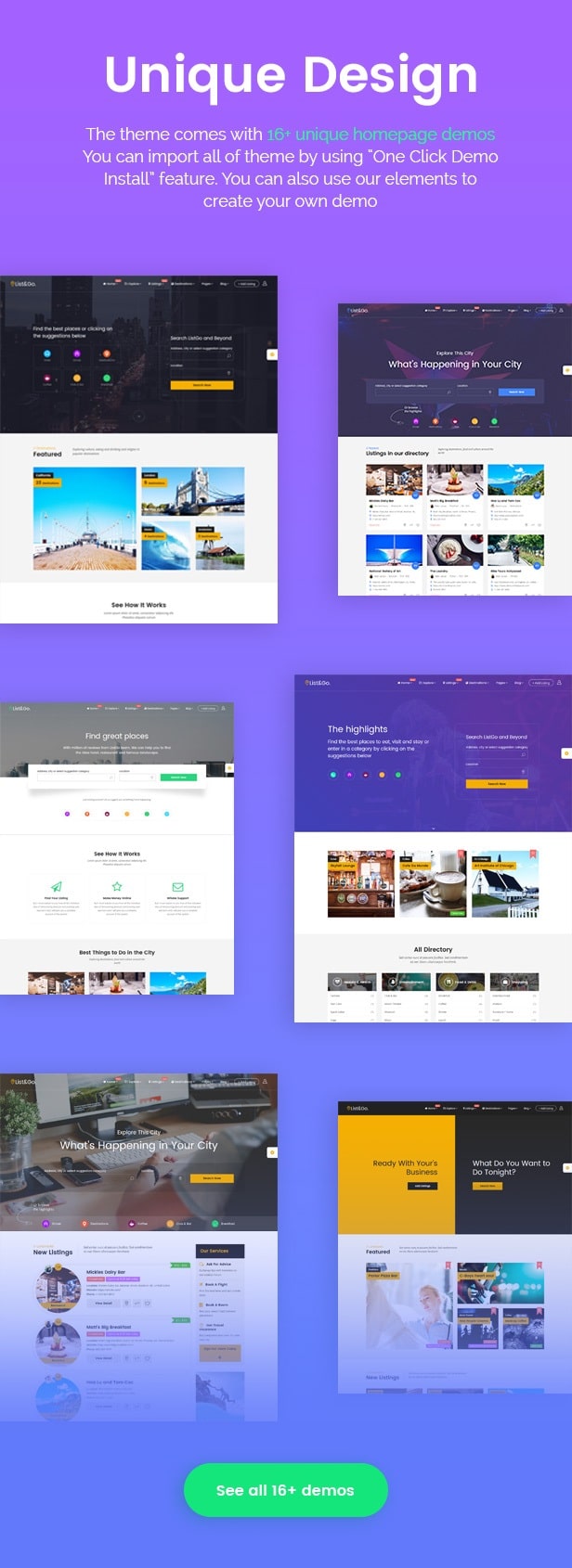The image features a blue background with white text at the top that reads "Unique Design" in bold. Below that, a lighter blue text states, "The theme comes with 16+ unique homepage demos." Further down, it is mentioned in white text that users can import all these themes using a "one click demo install" feature and also have the option to create their own demos with available elements.

The image then showcases six different demo layouts arranged in a 2x3 grid. The first demo, positioned at the top-left, has a dark background with a white bottom. The demo next to it has a dark blue background with a white bottom. The second row features a very light green with a white bottom on the left and a regular blue with a white bottom on the right. The third row begins with an image of an office setting on the left, followed by a yellow and black theme with a white bottom on the right. As the background color progresses downward, it becomes lighter.

At the bottom center of the image, there is a green rectangular button with rounded corners that appears to say "See All 16+ Demos" in white text, although it is slightly blurry and difficult to read.